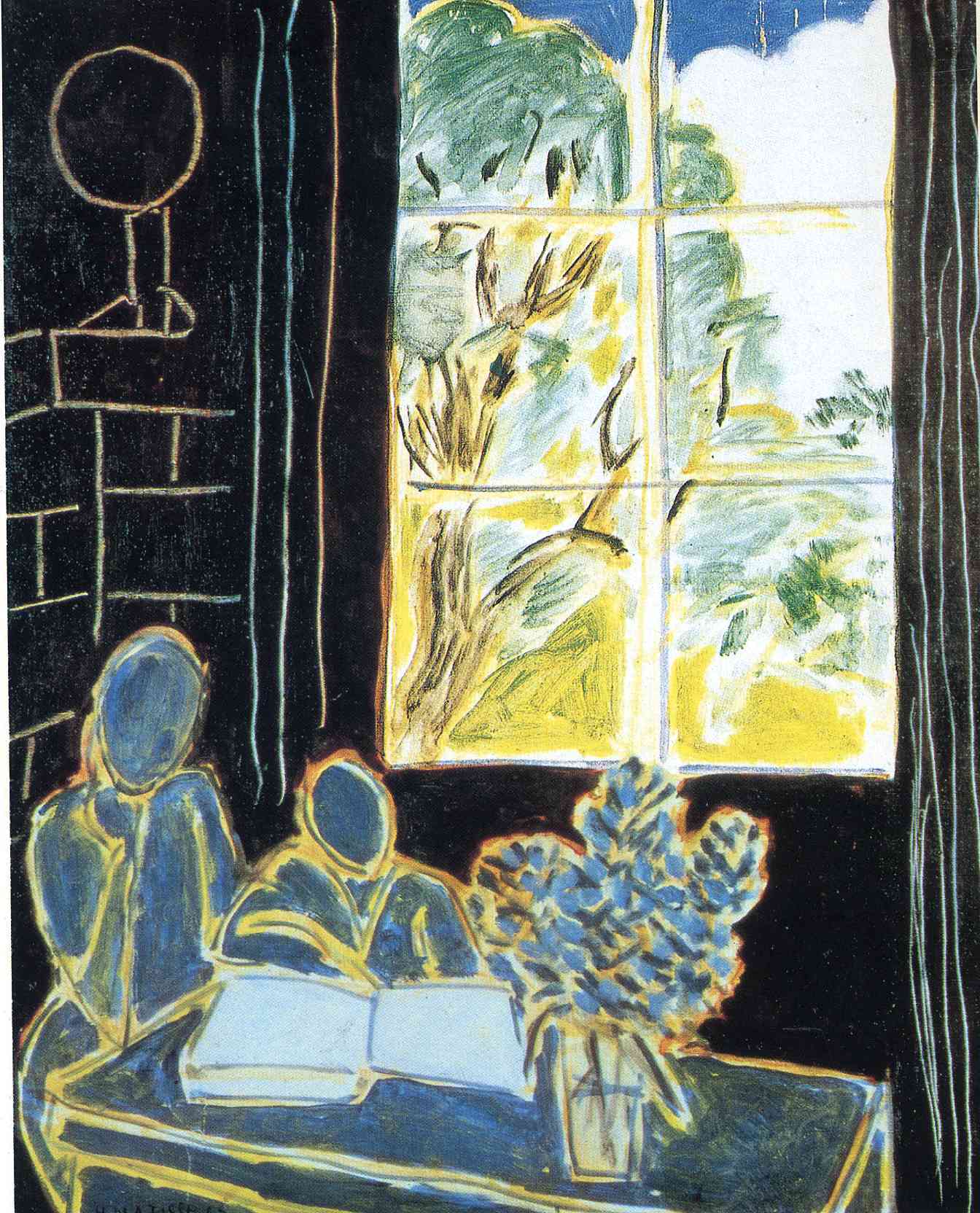In this impressionistic and abstract painting, the scene unfolds within a dimly lit room dominated by a black wall that suggests the presence of bricks. At the center of the composition, a table hosts a vivid depiction of two abstract figures, possibly a parent and child, engrossed in a book. Their forms are painted in muted tones of blue, yellow, and gray, blending seamlessly with the similarly colored table. Beside the book sits a glass or vase containing blue and gray flowers. The figures lack facial features, emphasizing their abstract nature.

In the background, a window framed by black curtains offers a glimpse into a contrastingly vibrant outdoor landscape. The sky is tinged with blue, dotted with clouds, and the scene includes impressionistic representations of trees with visible branches, yellow grass, and hints of green and brown. The colors outside, in stark opposition to the muted interior, radiate a lively, almost neon quality. The room itself, appearing almost as if the lights are off, casts the figures in a mysterious, shadowy light, further emphasizing the abstract and impressionistic style of the artwork.